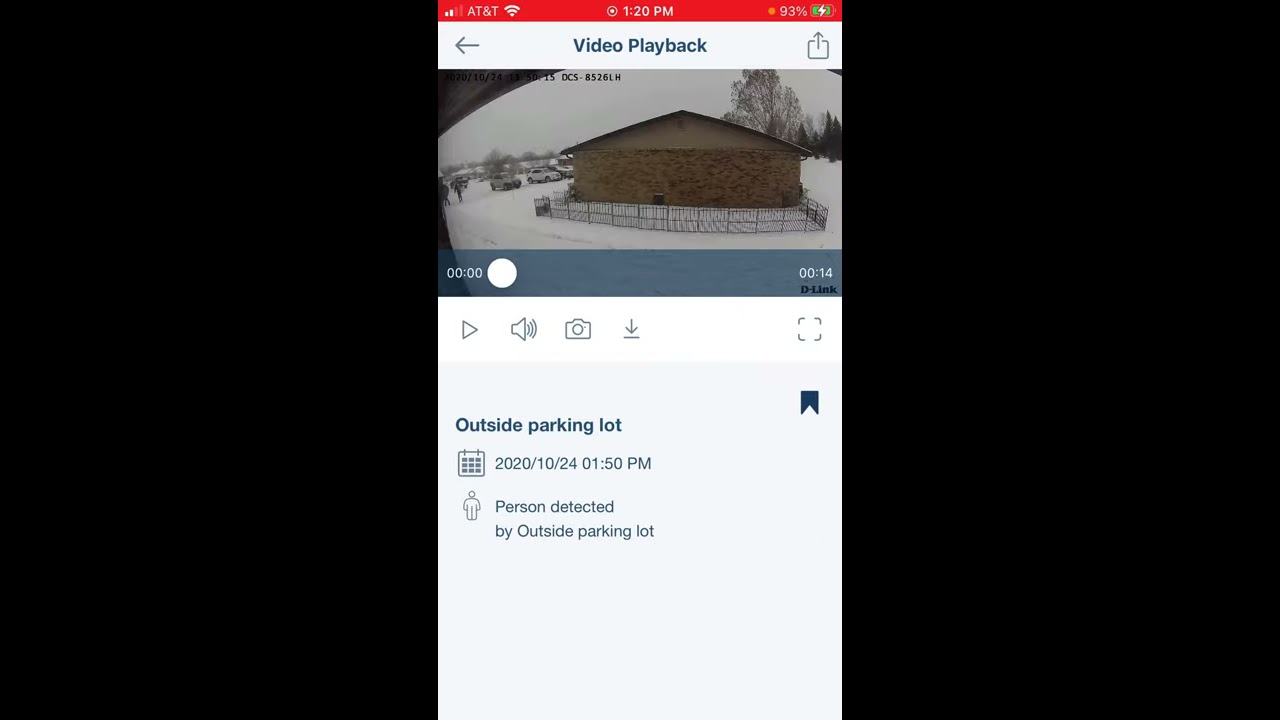The image is a screenshot from an iPhone displaying a Nest Cam video playback interface. The screen is divided into three parts, with black borders on the left and right and the central area containing details of the video playback. At the top, there are status indicators showing "AT&T," the time "1:20 p.m.," and a battery charge of "93%," all within a red border. Below this, blue text reads "video playback," accompanied by a back arrow and a send icon in white.

The main content of the screenshot features a security camera feed showing the side of a brick house with a tannish hue, surrounded by a wrought iron fence. The ground is covered in snow, and there are trees and cars visible in the background, indicating an outdoor, wintery setting. On the lower part of the video feed, it displays the timestamp "0:14" indicating 14 seconds into the video. Further below, text reads "outside parking lot 10/24/2020 1:50 p.m. person detected by outside parking lot," complemented by a drawn image of a person. This information implies that the security camera has detected a person in the specified area.